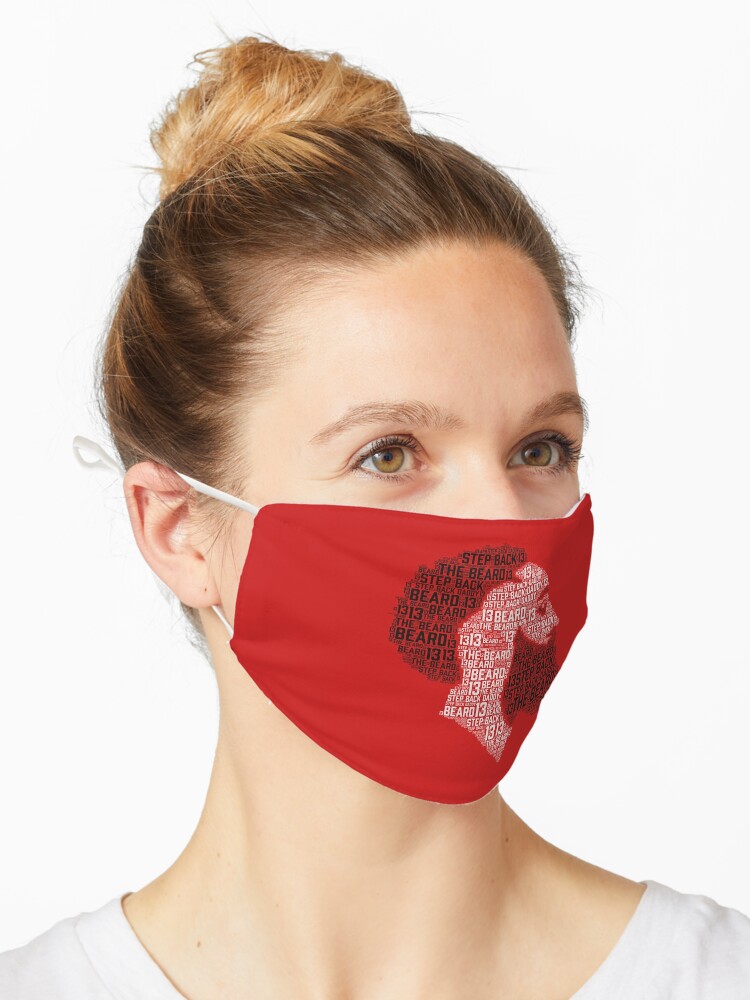This close-up portrait captures a middle-aged Caucasian woman with fair skin, beautifully light brown hazel eyes, and blonde hair styled in a swirly bun with a few tendrils escaping. She is looking off to the side at an upward angle, her gaze thoughtful. She wears a plain white crewneck t-shirt, and most prominently, a bright red face mask with white ear elastics—the kind often worn during the COVID-19 pandemic. The mask is adorned with an intricate design of Houston Rockets basketball player James Harden, constructed from black and white typographic elements. The black words form his hair and beard, featuring phrases like "step back," "13," and "beard," while the white words make up his skin and reiterate the same phrases. The background of the image is pure white, highlighting the woman’s contemplative expression and the detailed artwork of the mask.